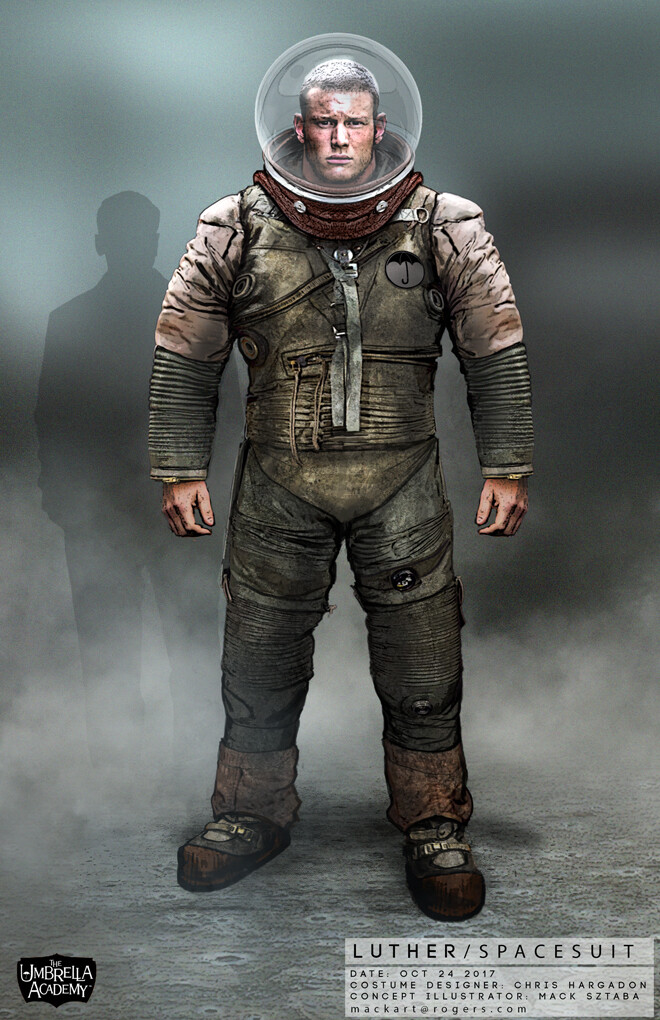This is a highly detailed digital or artistic image of Luther from the TV show "The Umbrella Academy," dated October 24, 2017. The piece, lacking a set border or background, is vertically rectangular and prominently features the silhouette of a man standing on a gray surface in the lower-left corner. Above him, gray splotches are visible, transitioning to a darker, blackish area in the upper and center right, with a misty white hue at the bottom.

Luther is depicted in a notable spacesuit, designed by Chris Hargadon, with concept illustration by Mac Sataba (email: macart at rogers.com). The spacesuit is distinctive with a fishbowl-type helmet, large shoes, and several hefty metal parts on the arms and stomach, indicative of a suit weighing several hundred pounds. Unique elements include the absence of gloves on Luther and the extensive detailing that captures the bulkiness and industrial design of the suit. The bottom right of the image contains the text “Luther Spacesuit” along with the metadata, while the bottom left displays the logo of “The Umbrella Academy.” This show features children with superpowers, born on the same day to mothers who suddenly became pregnant, with Luther's abilities involving a super-strong, part-ape, part-human physiology.